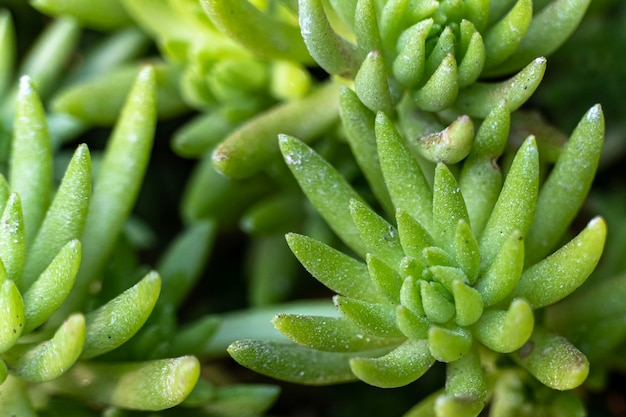This image is a highly detailed close-up of a succulent plant with distinctive characteristics. The photo captures cone-shaped, thick leaves typical of succulents, arranged in a way that creates an almost flower-like shape. This floral pattern is more pronounced in the lower and upper right-hand parts of the image. The background is stark black, making the lime-green leaves stand out remarkably. Upon close inspection, the leaves reveal white and black speckling, resembling scattered white sugar. The succulent appears in a spiral formation, and individual stems become tighter and thicker as they converge toward the center. There are about five sections of these plants visible in the photograph, each with their lime-green leaves tipped with white, adding to the intricate texture and visual appeal.